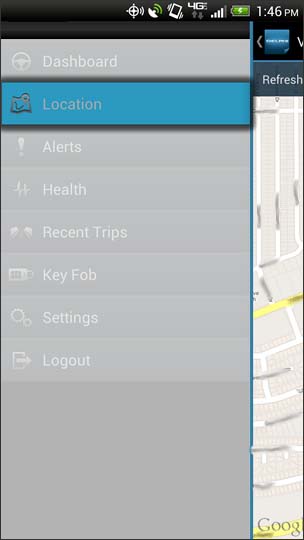The image depicts a cell phone screen at 1:46 p.m., as indicated by the green battery icon. The status bar at the top is black and shows that the phone is on vibrate mode, connected to a 4G network with full cell bars, and currently charging. 

A gray pull-out menu from the left, featuring white text, is partially covering a Google Map. The menu has the following options listed from top to bottom: "Dashboard," "Location," "Alerts," "Health," "Recent Trips," "Key Fob Settings," and "Log Out." The "Location" option is highlighted in blue. 

Due to the menu's intrusion, only a narrow strip on the right side of the map is visible. The map, marked with yellow patches and predominantly light gray or white tones with some black areas, appears to have blurred street names. The bottom of the map has the "Google" watermark, confirming it as a Google Maps interface. 

The color palette in the image includes gray for the menu background, white for text and elements of the map, blue for the highlighted option, yellow for certain map areas, and black for the map background and other details. No specific website or additional identifying information is present on the screen.